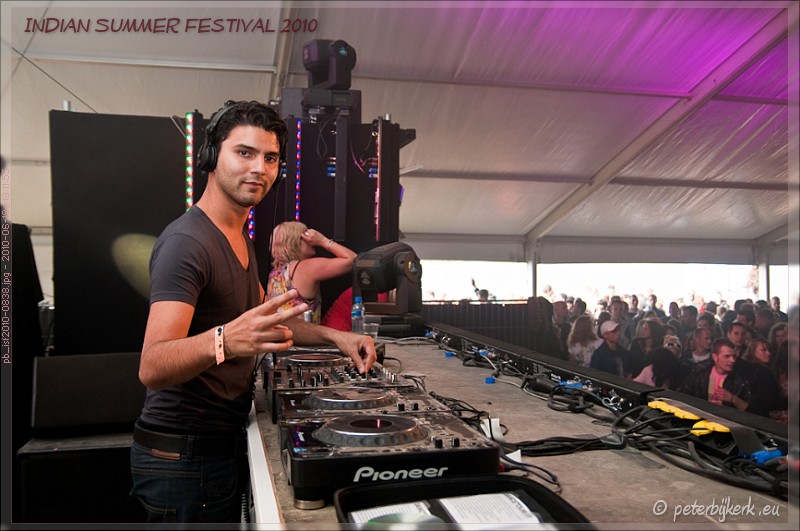The image depicts a lively scene at the Indian Summer Festival 2010, featuring a DJ positioned on a platform inside a large canopy-like tent with a white ceiling supported by poles. The male DJ, with an olive skin tone, is front and center, wearing a grey V-neck T-shirt, blue jeans, and a brown belt, with black headphones on. He’s looking directly at the camera, flashing a peace sign with his right hand. His DJ station is equipped with multiple turntables and mixers, prominently displaying the Pioneer brand. Surrounding the platform are large speakers with additional tall speakers set on the platform. In the crowd below, which is filled with enthusiastic festival-goers dancing and enjoying the music, a woman with blonde hair and a pale skin tone can be seen near the DJ, looking out into the crowd. The photo also notes a copyright “peterbizjerkkirk.eu” at the bottom left-hand side.